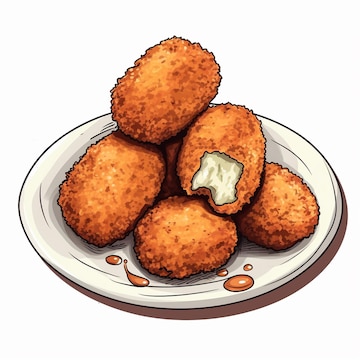This digitally created, cartoon-like image features five small, breaded food items arranged on a white, ceramic plate. These fried nuggets, brown and crispy on the outside, have a white filling visible where one piece has been bitten into, suggesting a cheese or chicken interior. The items appear greasy, with drops of a brown liquid scattered around the plate. Shadows under the plate further enhance the hand-drawn, animated depiction of this appetizing scene.